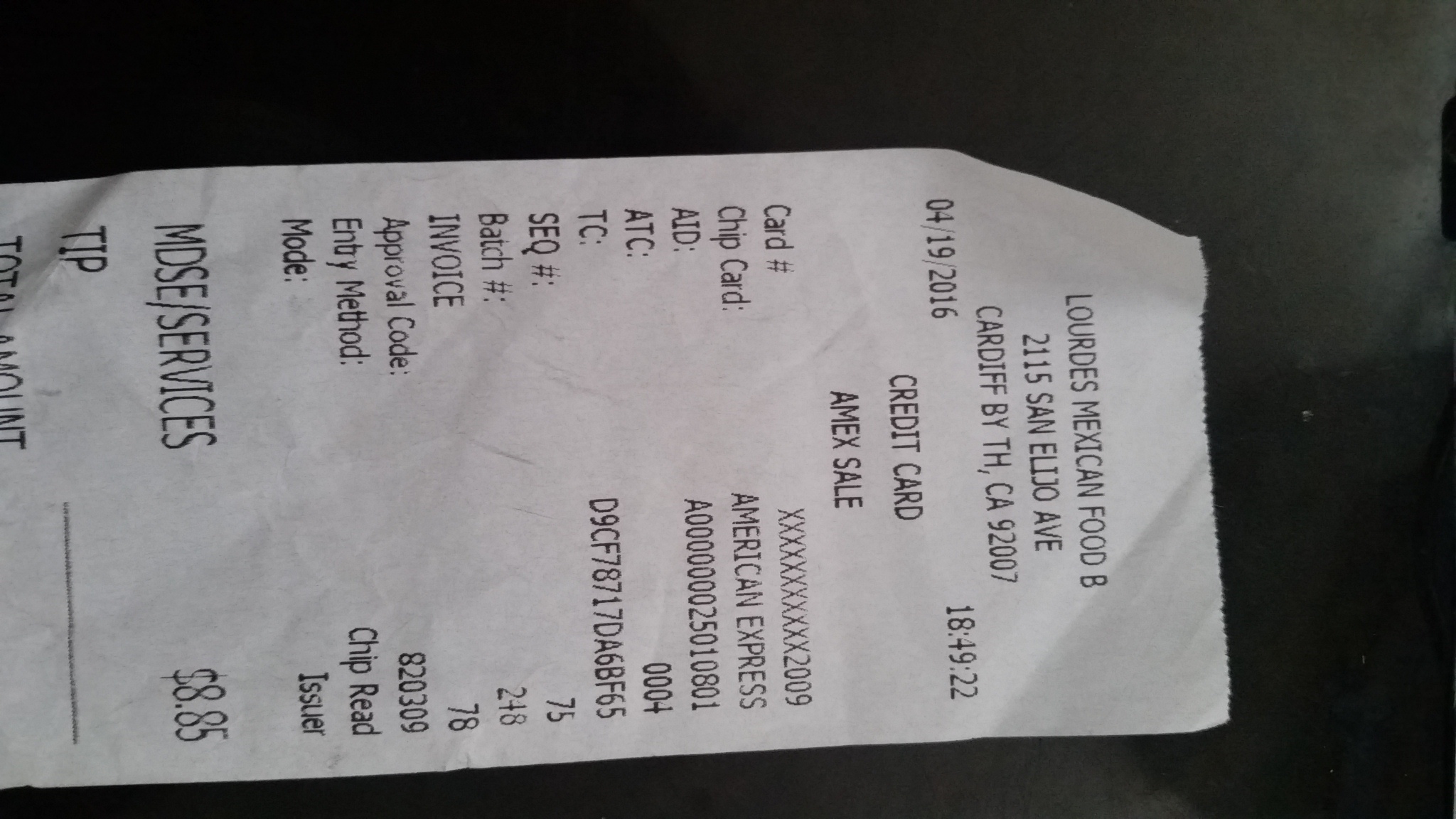The image depicts a detailed color photograph of an old-fashioned white paper register receipt, positioned sideways on a black surface. At the top, the receipt shows the business name "Lourdes Mexican Food," located at "2115 San Elijo Avenue, Cardiff, CA 92007." The transaction date is April 19, 2016, and it indicates a credit card payment, specifically an American Express card. Additional details include card number entries, chip card information, and various invoice identifiers. The total cost for the meal, listed as merchandise/services, amounts to $8.85. The receipt is printed in black ink, and there is no tip amount filled in. The word "total amount" is visible at the bottom, emphasizing the final charge.